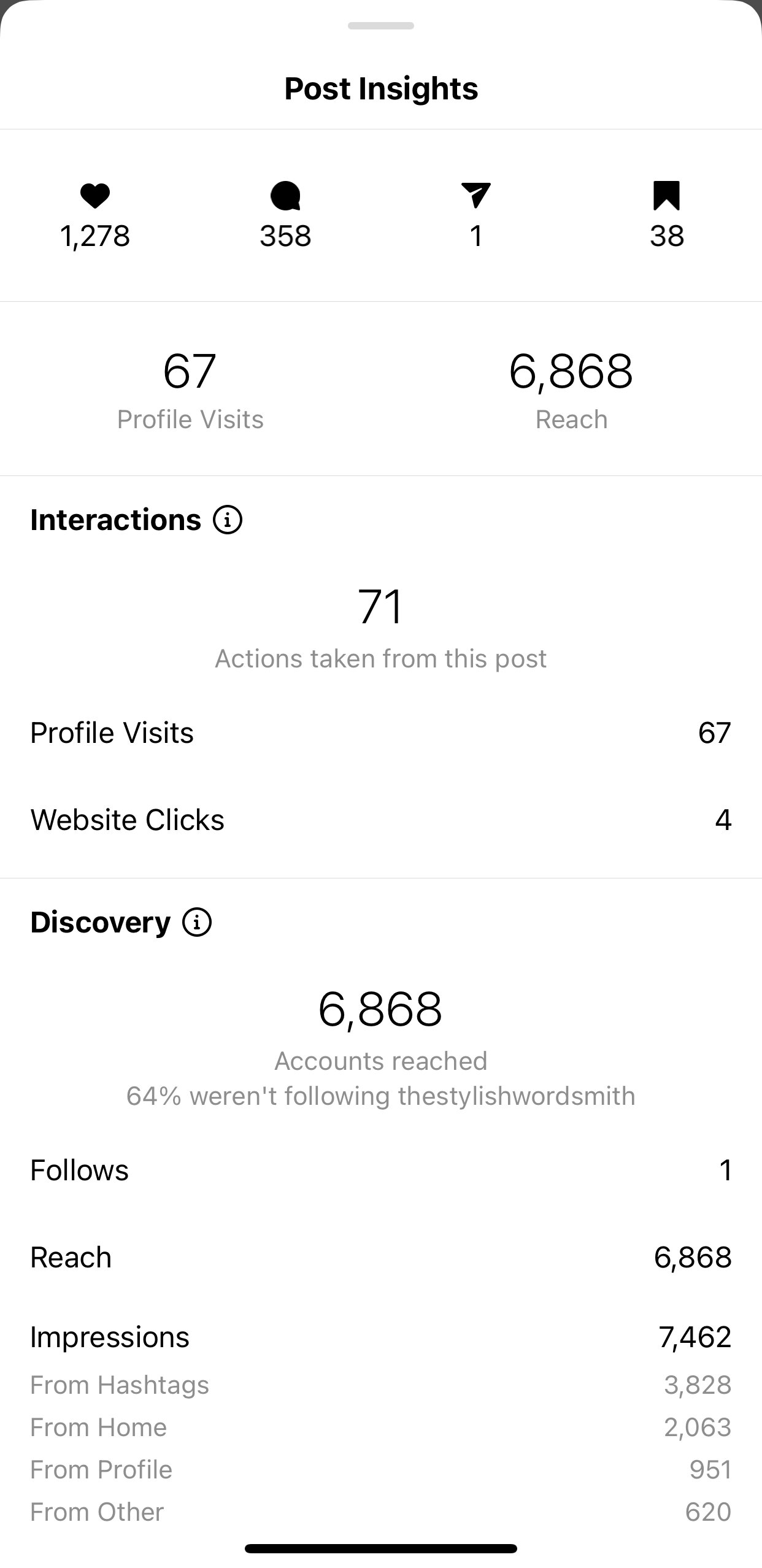Screenshot of mobile app menu features a detailed analytics breakdown of a social media post. The interface is designed with a white background and uses black font for text clarity. At the top, the heading "Post Insights" is displayed, followed by a thin gray horizontal line. Below this line, various engagement metrics are listed:

- Heart icon: 1,278
- Comment icon: 358
- Shares icon: 1
- Bookmarks icon: 38
- Profile visits: 67
- Reach: 6,868

Further down, under the section "Interactions," it details:

- Actions taken from this post: 71
- Profile visits: 67
- Website clicks: 4

The next section, "Discovery," outlines:

- Accounts reached: 6,868 (with 64% being followers of "The Stylish Wordsmith")
- Follows: 1
- Impressions: 7,462
  - From hashtags: 3,828
  - From home: 2,063
  - From profile: 951
  - From other sources: 620

A black line separates these sections. The top part of the image with the hearts, comments, shares, and bookmark counts includes small corresponding icons next to each metric.